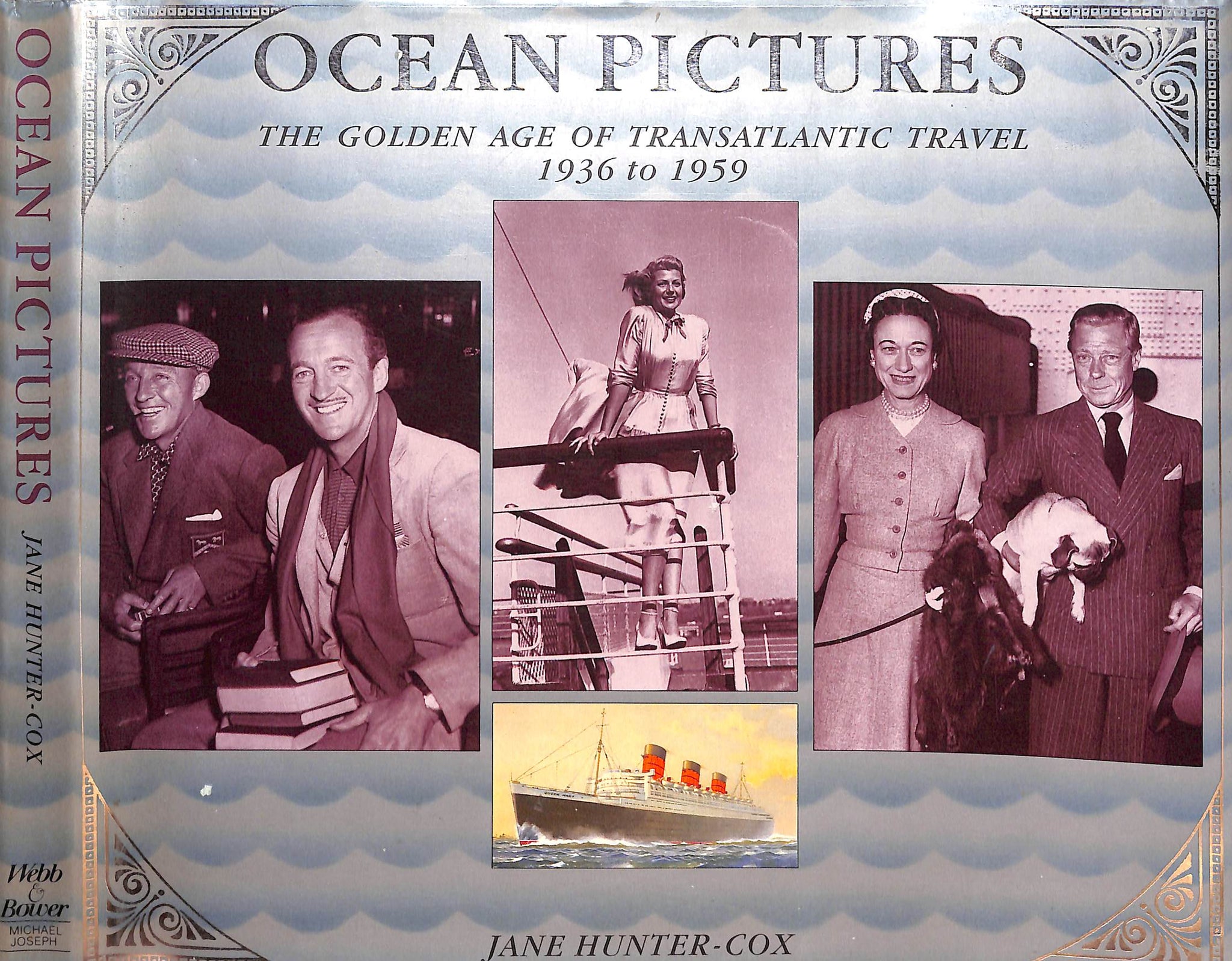This is an image of a book cover titled "Ocean Pictures: The Golden Age of Transatlantic Travel 1936 to 1959" by Jane Hunter Cox. Spanning a blue wave-patterned background, the cover features ornate curlicues in the corners and is slightly bent to reveal the spine, which also reads "Ocean Pictures, Jane Hunter-Cox, Weber and Bauer, and Michael Joseph."

The cover showcases three main images prominently across its middle. On the left, two gentlemen are seated: one with a mustache, wearing a suit jacket, a button-up shirt, a watch on his left wrist, and holding a pile of books on his lap, while the other sports a fedora cap and jacket with a handkerchief peeking out. The central image depicts a woman standing on the bowspit of a ship, her white dress with many buttons flying in the wind, her hair and skirt streaming back, and wearing high-heeled, strapped sandals. The right-hand picture shows an older couple; the man in a pinstripe suit with a tie is holding a small dog, while the woman, adorned in a hat, pearls, earrings, a buttoned-up jacket, and carrying a fur coat over her left arm, is managing the dog’s leash.

Beneath the central image is a fourth smaller illustration of a ship sailing on rough seas, oriented toward the left on a yellow background. The detailed depiction evokes the essence of the golden age of transatlantic travel, capturing the elegance and allure of the era through its richly detailed imagery.